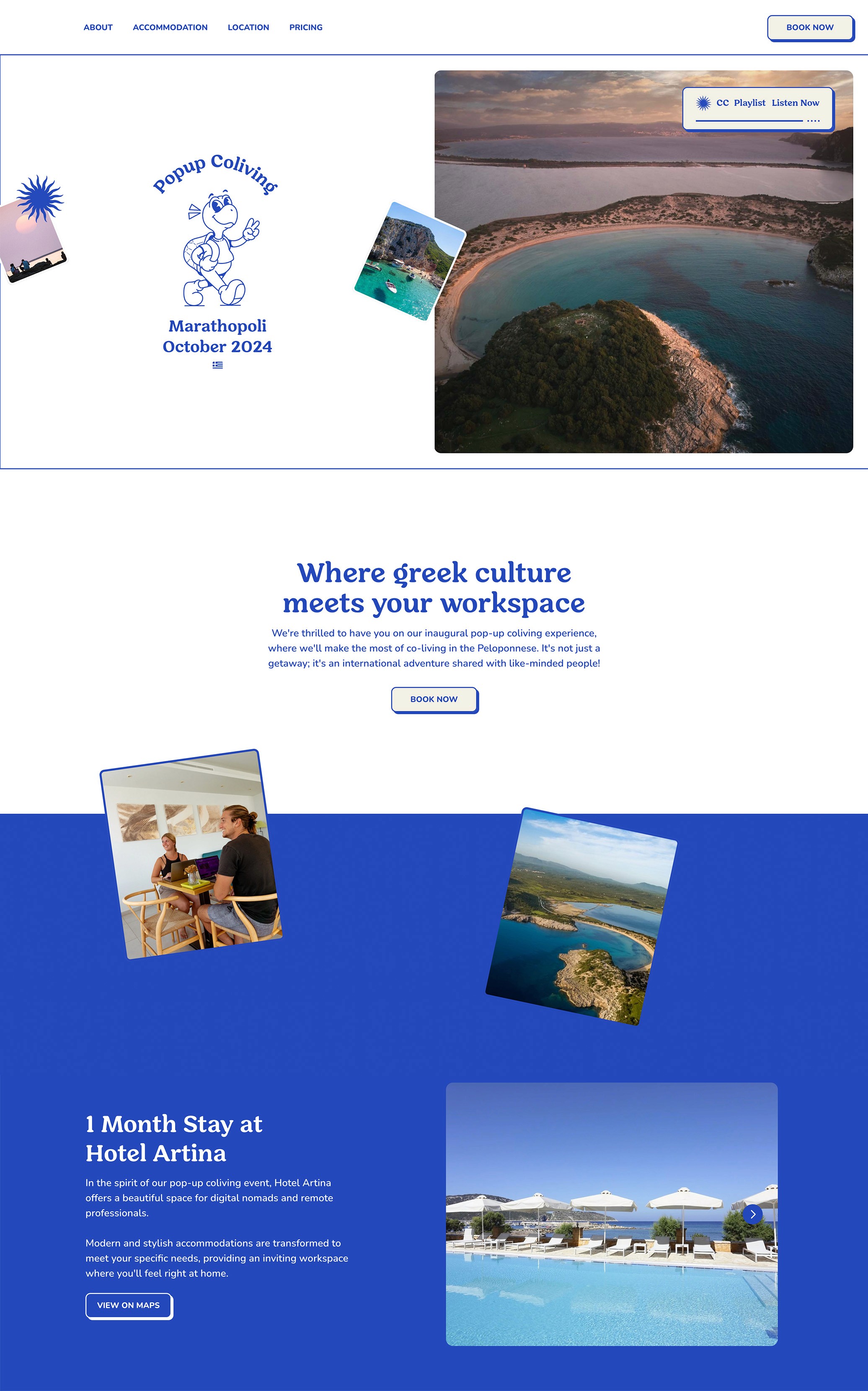The image is a rectangular travel poster for a pop-up co-living experience in "Marseipoli" (or similar name), taking place in October 2024. The poster emphasizes the fusion of Greek culture and a modern workspace environment. At the top, there is a charming cartoon turtle with the text "Marseipoli, October 2024," alongside a photograph of a scenic crater lake or bay. Beneath this, there's the tagline "Where Greek Culture Meets Your Workspace" with an invitation to book now, and some smaller, illegible text.

The poster is divided into two main visual sections: 

1. The upper section features the scenic photograph of the crater lake and the enticing slogan mentioned above. 
2. The lower section, set against a blue background, displays several photographs: a pool with lawn chairs, lounge chairs, and white umbrellas; a man with a ponytail; a woman seated at a table in a relaxed setting; and a mountain lake or bay from an aerial view. This section promotes "One Month Stay at Hotel Artina," accompanied by welcoming text about the inaugural pop-up co-living experience and additional unreadable small print.

Overall, the detailed imagery and text aim to attract participants to an immersive, culturally rich accommodation experience blending leisure and work.